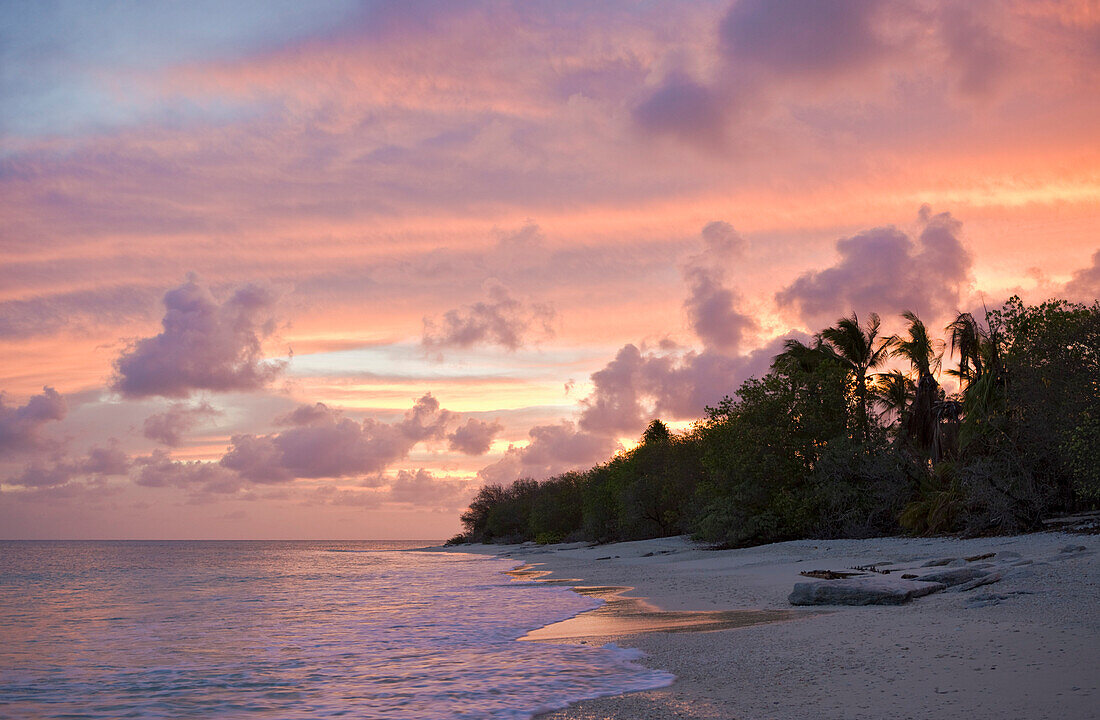The photograph showcases a serene beach at sunset, where the incoming tide gently caresses the shoreline. Dominating the bottom right corner is a stretch of typical brown beach sand, sparsely populated with indistinct objects that could be rocks. The beach line starts at the bottom middle, curves slightly upward to the left, and eventually leads to an area rich with short, stout trees. Behind them lies a dense assemblage of taller trees that extend from the right towards the middle of the image, shrinking as they vanish into the horizon close to the water's edge.

On the left side of the image, waves roll in, exhibiting a frothy white crest as they blend with the pinkish-hued water reflecting the sunset's colors. Above the central horizon, the sky transitions from clear blue in the upper left to an array of purples, grays, and soft oranges. To the right, patches of yellow show through the orange-tinged clouds, suggesting the hidden sun's glow. The sky dominates the top two-thirds of the image, with more blue patches peeking through the gray clouds on the left.

Overall, the scene is a calm depiction of a beach evening, marked by its vibrant yet soft sunset tones, the encapsulating embrace of the colorful sky, and the quiet dignity of the distant trees with their mirrored shadows in the tranquil water below.